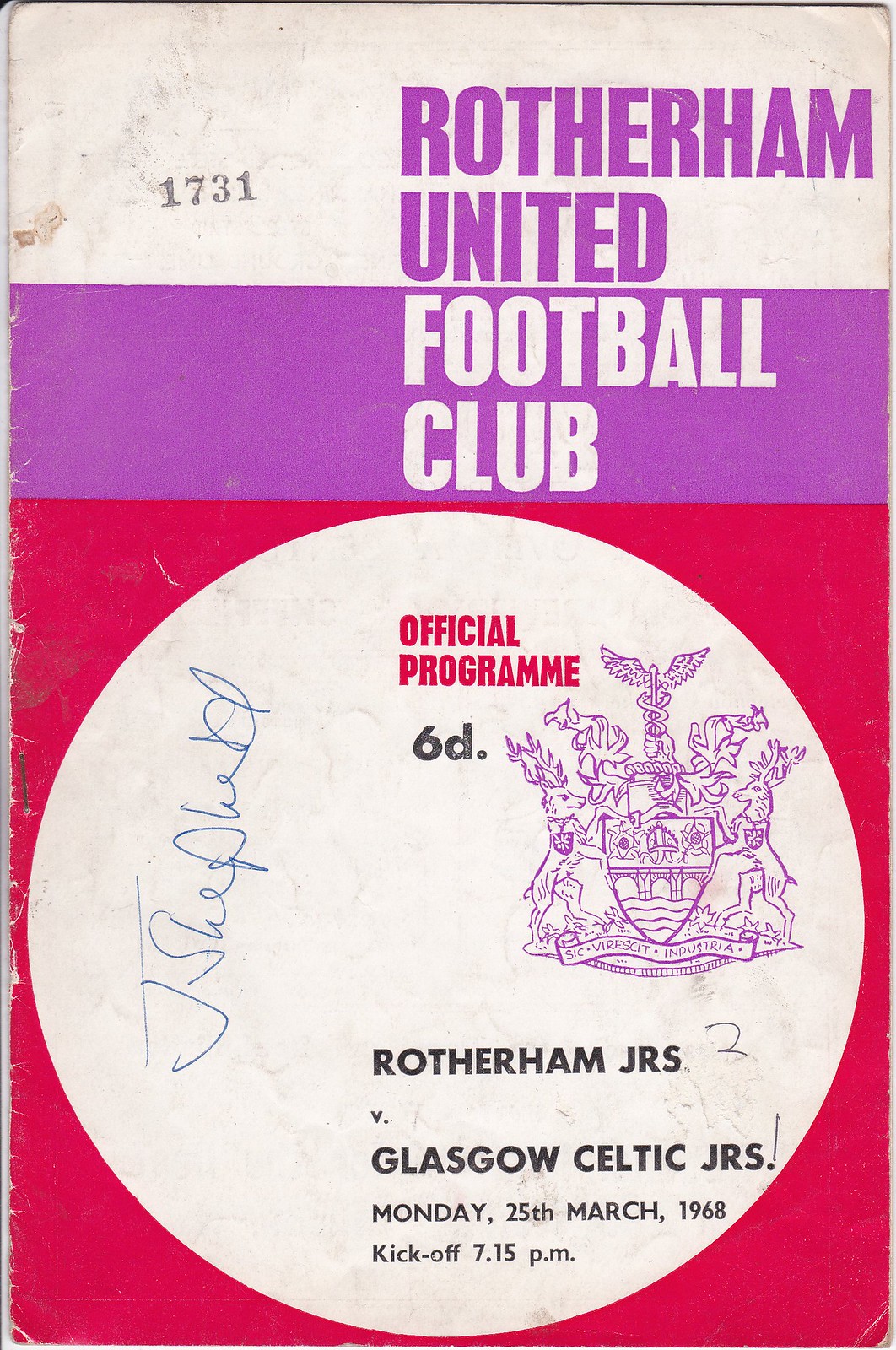This image displays an old program for a soccer match by Rotherham United Football Club. At the top, the page is white, featuring the text "Rotherham United" in purple letters. Beneath that, a purple stripe bears the words "Football Club" in white text. The bottom section of the program is red, with a prominent white circle containing the text "Official Program" in red. Below this, it states "6D" and provides the match details: "Rotherham JRS v Glasgow Celtic JRS, Monday 25th March 1968, kickoff 7.15 p.m." Within the white circle, there is a purple emblem resembling a shield flanked by two deer. Additionally, to the left of the circle on the red background, there appears to be a blue ink signature, possibly from a player, which looks like it says "Jay Shepard."